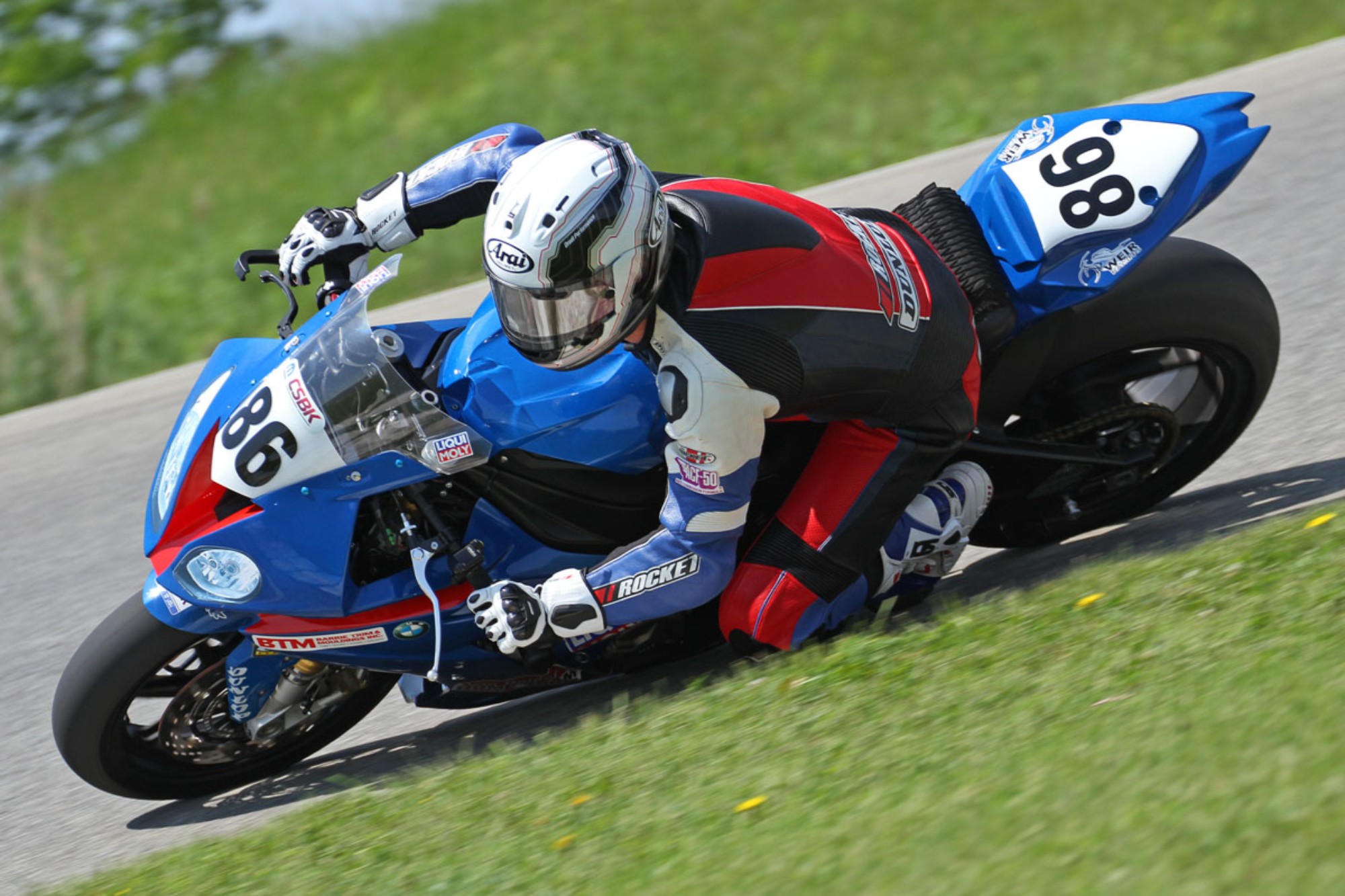The image depicts a motorcycle racer making an extremely sharp turn on a racetrack. The rider, who is practically touching the ground due to the sharp angle, is dressed in a full-body leather jumpsuit with white, blue, black, and red accents. White gloves and a white and black helmet complete his gear. His blue and red motorcycle, marked with the number 86, also features a few partially obscured logos, including one for Dunlop. The photograph is zoomed in, emphasizing the intensity of the turn, with no other bikes in sight. The backdrop consists of asphalt and surrounding green grass, highlighting the solitary focus of the rider as he leans deeply into the curve.